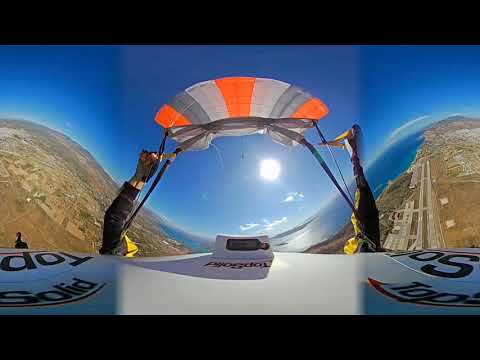The photograph captures an outdoor, daytime scene viewed from a high vantage point, possibly mounted on a paragliding or hang gliding apparatus. The image is framed by black bars at the top and bottom, adding contrast to the vibrant depiction. The scene is heavily distorted, giving it a wave-like appearance, with the ground rising on the left, dipping into a u-shape in the center, and rising again on the right. The sky is a brilliant, deep blue with a couple of scattered clouds, and a white sun is visible in the middle, reflecting off the terrain.

At the bottom of the image, a white component is visible with black writing that reads "TOP" and "SOLID." This object also has a digital device, possibly a screen, at its tip. Two arms, adorned in long-sleeved jackets, extend upward, gripping a support structure. The glider or parachute-like canopy above is striped in orange, gray, and white.

The view below reveals brown terrain with what appears to be a landing strip to the right and some waterbody separated from the sky, stretching into the background. Urban elements such as streets and buildings appear distant and warped due to the camera's lens effect. The overall composition vividly conveys the sensation of a high-altitude flight, with the expansive landscape and sky offering a breathtaking, albeit distorted, panorama.